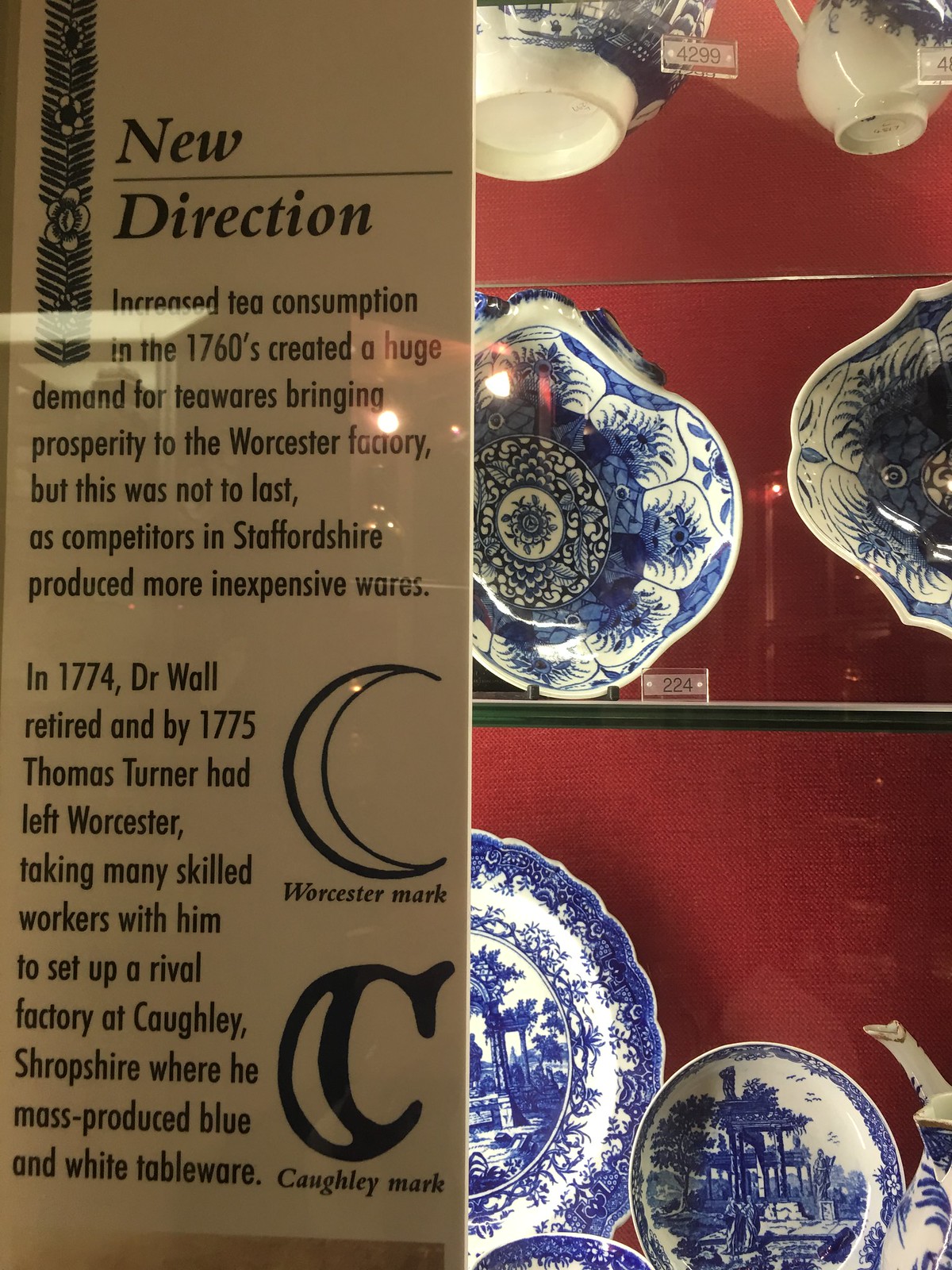In the photograph, we see a museum exhibit that features a meticulously arranged display of blue and white crockery items set against a vibrant dark red background. The exhibit showcases a range of teaware, including ornately decorated plates, bowls, and teacups, each adorned with various intricate designs such as flowers, houses, and trees. These pieces are systematically placed on glass shelving and are identified by number plaques, like the one marked 224.

On the left side of the image, there is a vertically oriented, rectangular information board made of light brown material. The board features a title in bold black letters at the top that reads "New Direction." Beneath the title, the board explains how increased tea consumption in the 1760s created significant demand for teawares, bringing prosperity to the Worcester factory. However, it notes that this boom was short-lived due to competition from Staffordshire, which produced more affordable wares. The text further details that Dr. Wall retired in 1774, leading to the departure of Thomas Turner and many skilled workers who set up a rival factory in Caughley, Shropshire, where they mass-produced blue and white tableware. The board also includes symbols representing the Worcester and Caughley marks, with the former resembling a crescent moon and the latter a thicker, C-shaped mark.

Overall, the image captures a rich historical narrative and beautifully showcases the craftsmanship of 18th-century teawares.